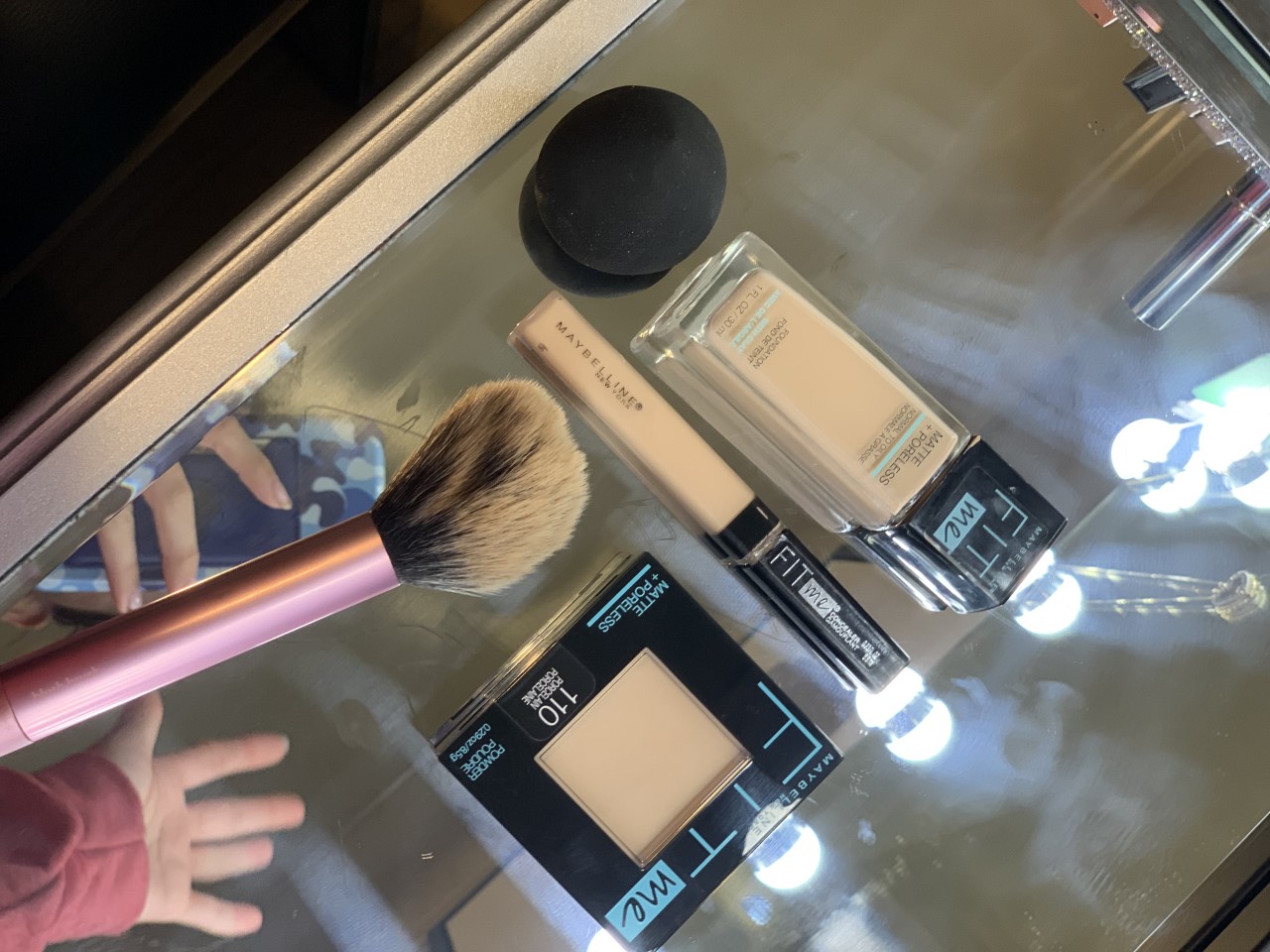The image depicts a glass tray viewed from an upside-down perspective. The tray's center is made of clear glass, while the edges are framed in a luxurious gold hue. A reflection of someone’s right hand, clad in a pink sweatshirt, is visible in the bottom left corner, providing a focal point for the scene. Above this hand's reflection, fingers holding a blue object can be discerned.

Off the tray's left corner, an angled makeup brush with a pink barrel and a fluffy bristle head extends into view. Dominating the top-middle portion of the photograph, a black circular sponge sits prominently, hinting at its utility in makeup application. Directly beneath the sponge, a bottle of foundation rests, with its glass body filled with a tan liquid and capped with a black lid labeled "Fit Me." The bottle's cap points downwards, adding a sense of orientation to the image.

To the left of the foundation bottle, a tube of concealer is placed horizontally. The concealer features "Maybelline" written at its base and "Fit Me" on its black cap. Further left, a compact powder case with a black exterior and a transparent center displays the light brown powder within. The case is marked with "110" at the bottom and "Maybelline Fit Me" across the top, succinctly identifying its brand and shade. Together, these items form a carefully arranged still life of personal grooming essentials, reflected elegantly on the glass tray.